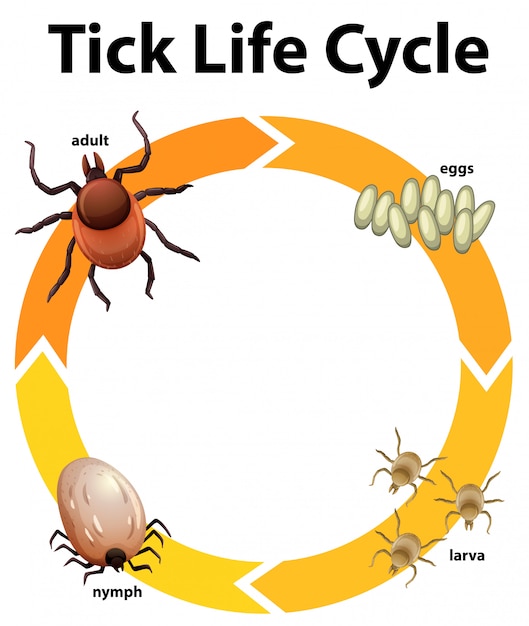The illustration, titled "Tick Life Cycle," is a detailed and colorful infographic commonly found in biology or science textbooks. The title is rendered in black uppercase and lowercase letters. The main feature is a circular diagram shaded in hues of gold, orange, light orange, and dark gold. The cycle begins at the top left with an illustration of an adult tick and flows counterclockwise.

Next to the word "eggs" are several oval egg shapes, depicted in the top left section. From there, the cycle progresses to the bottom right, showing three small larval ticks. The following stage, positioned at the bottom left, portrays a single nymph tick, which is slightly larger than the larva. Finally, the cycle returns to the top left with another image of an adult tick, completing the loop.

Each phase of the tick's development—from egg, larva, nymph to adult—is clearly marked with text and illustrations. Arrows connect each stage, highlighting the continuous nature of the life cycle, which repeats as the adult tick lays more eggs. The diagram serves to educate on how ticks develop and the process by which they may potentially spread infections to humans and animals, such as canines and cats.